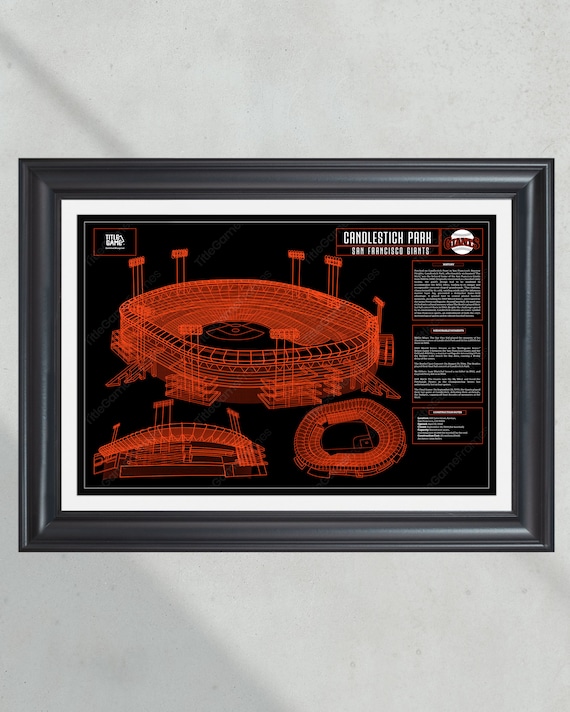This image showcases a framed, three-dimensional line drawing of Candlestick Park, encased in a black frame and mounted on a gray wall. The artwork, which resembles a blueprint or a 3D model, is vividly illustrated in a bright to medium red hue against a dark background. Titled "Candlestick Park," the print prominently features the San Francisco Giants' logo—a baseball with “Giants” written in black text—situated in the upper right corner, along with the team name in large white letters. 

The detailed diagram includes three vantage points of the stadium. The first view is an aerial perspective that captures the full exterior shape of the stadium, including the infield and lighting fixtures. The second angle provides a ground-level, tilted view that showcases the stadium's flowing curves. The third perspective, taken from a high angle above, clearly displays the entire outfield and the arrangement of seating areas. Due to the fine details and small text within each section, some elements are difficult to read from a distance, yet the overall representation vividly captures the architectural essence of Candlestick Park, emphasizing its role as a venue for the San Francisco Giants.